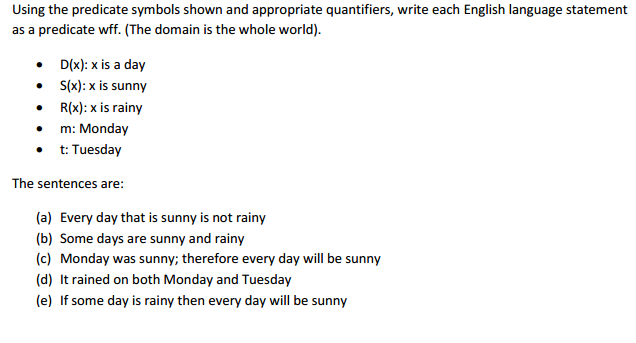The image features a plain white background with black text, presenting instructions and a series of logical statements formatted as predicate well-formed formulas (WFFs) in a bulleted list. The domain for these statements encompasses the entire world. The list includes the following predicates:
- \(D(X)\): \(X\) is a day.
- \(S(X)\): \(X\) is sunny.
- \(R(X)\): \(X\) is rainy.
- \(M\): Monday.
- \(T\): Tuesday.

The bulleted statements to be formulated into predicate WFFs are:
A. Every day that is sunny is not rainy.
B. Some days are both sunny and rainy.
C. Monday was sunny; therefore, every day will be sunny.
D. It rained on both Monday and Tuesday.
E. If any day is rainy, then every day will be sunny.

The text appears to resemble content typically found on a test or an online assignment, lacking specific details about its source or context.